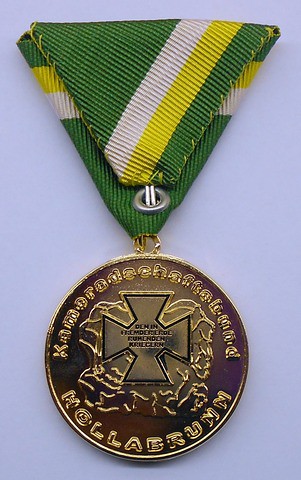This is a detailed close-up photograph of a military service medal and ribbon. The medal itself, resembling the size of a large coin, is golden or brass in color and features an iron cross at its center. The cross has intricate etchings, possibly a map, with black lettering that's tough to decipher, including portions that might read "Dem in" and "Rundlich-Killgern." Surrounding the cross, the inside edge of the medal features raised letters that appear to spell "Kameradenhafenbude" on the upper edge and either "Kallenbrun" or "Hollenbrun" on the lower circular edge. The cross is outlined in black, with what look like electrical patterns emanating from it.

The medal is suspended from a fabric ribbon, which forms an inverted triangle with its point connecting to the medal. The ribbon has an army green background with white and yellow diagonal stripes. The background of the image is lilac-colored, providing a subtle contrast to the medal and ribbon. Overall, the origin of this military ribbon and medal is unclear, lacking any distinctive markers that would indicate its country of origin.